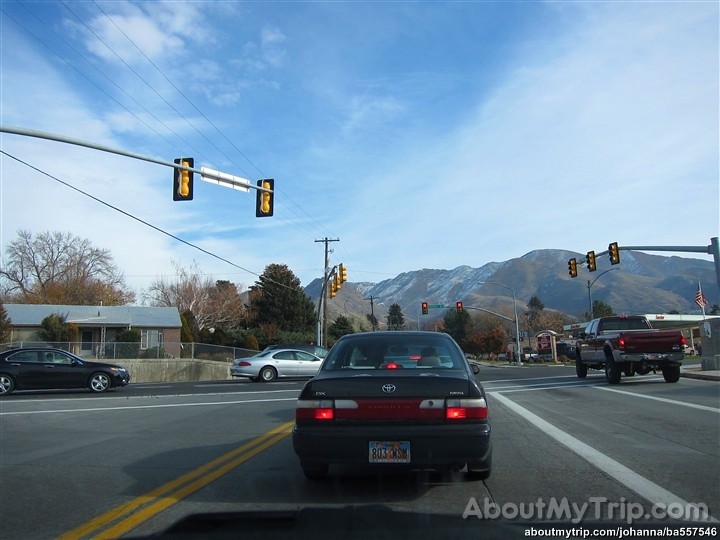Captured on a bright blue sunny day adorned with scattered white clouds, this photograph highlights a scene brimming with detail. Taken from inside a vehicle, the image centers on a black Toyota Corolla with a colorful license plate featuring blues and reds. The Corolla is positioned at a stoplight, easily identifiable by the yellow center line of the road and the red traffic light. To the right, a pickup truck waits patiently at the same intersection. In the background, a building with a white roof, likely a gas station, proudly displays a United States flag. The bottom right-hand corner of the photograph is marked with "aboutmytrip.com," indicating its source.